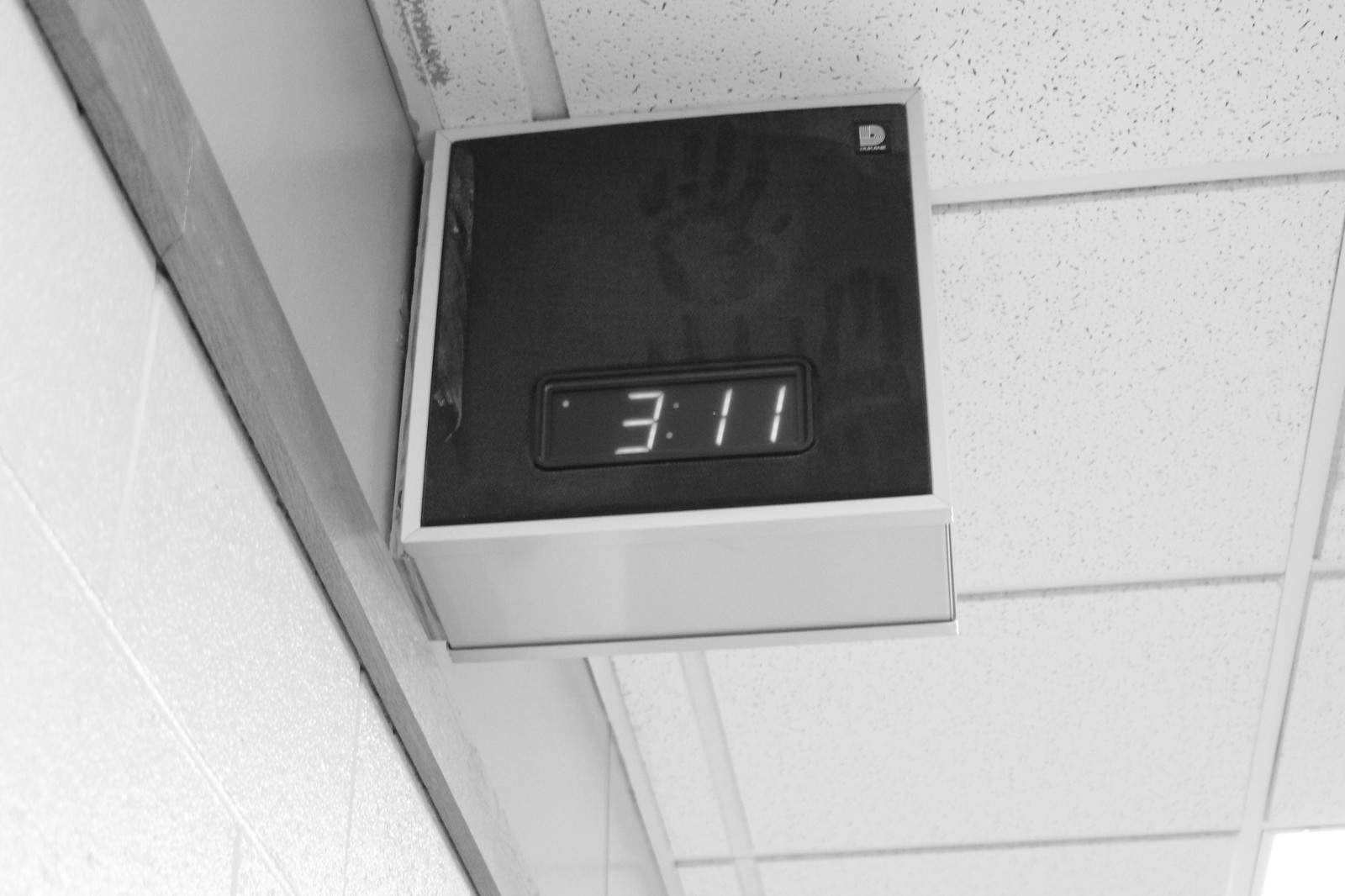In this striking black and white photograph, a digital clock displaying the time 3:11 is prominently featured. The grainy monochromatic tones lend a timeless quality to the scene. The clock is mounted on a white tile ceiling, its sleek surface marred by three small handprints, likely left by playful children jumping up to touch it. The handprints are faint but visible, their smudged outlines adding an element of human presence and curiosity to the otherwise sterile and uniform ceiling. The juxtaposition of the digital clock and the tiny, almost ghostly handprints evokes a sense of innocence and mischief within a structured environment.